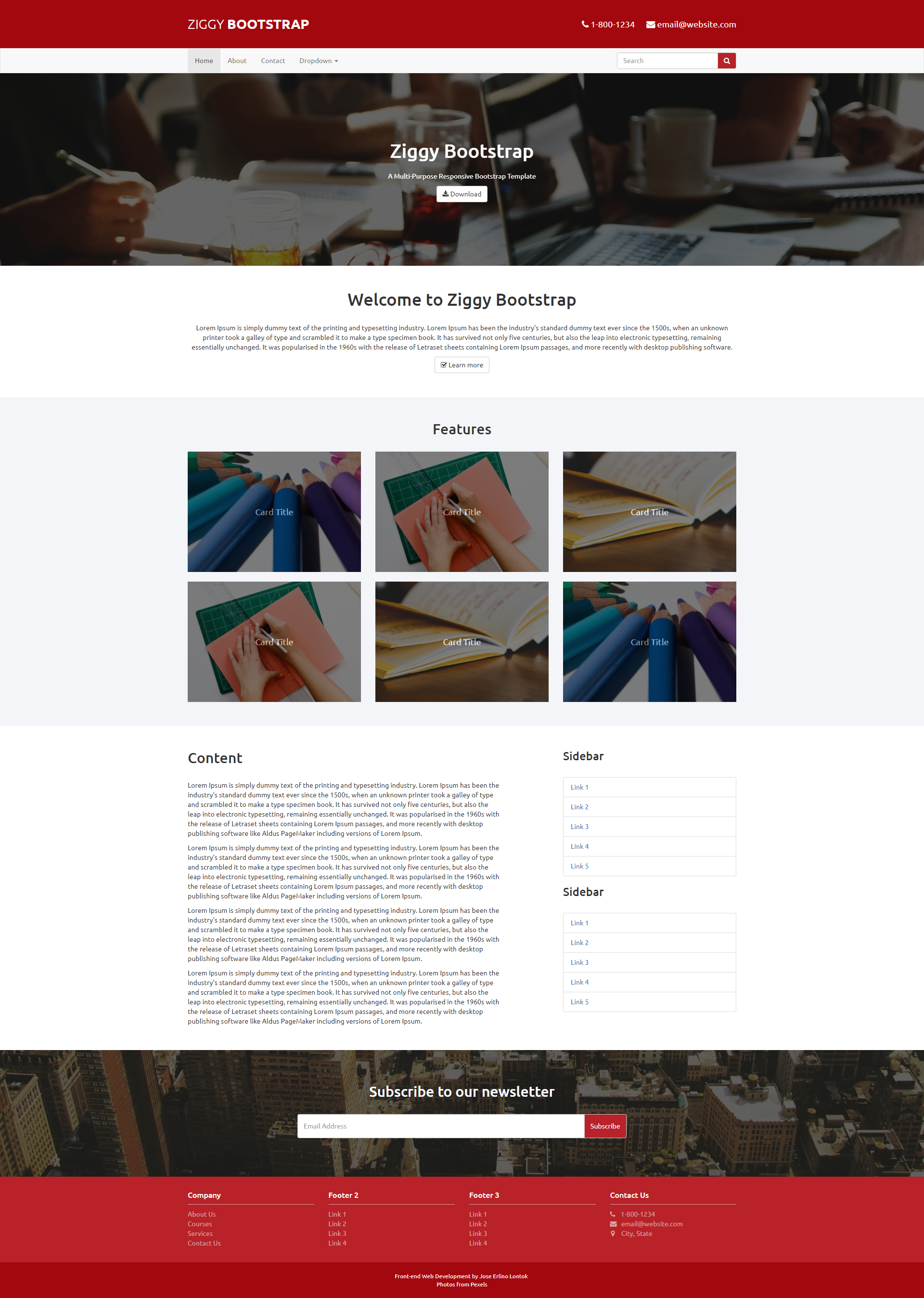This is a detailed photo of the Ziggy Bootstrap website, showcasing its dynamic and visually engaging layout. The website appears quite busy with several distinct sections. The color scheme prominently features shades of red, white, black, and blue, which gives the site a striking and professional aesthetic.

At the top of the page, the name "Ziggy Bootstrap" is prominently displayed, adding to the overall branding. The welcoming message, "Welcome to Ziggy Bootstrap," is prominently shown in bold black lettering towards the middle of the page.

Multiple images are used throughout the site, some of which are repeated. These images include close-up shots of turquoise and blue pencils arranged in a circular pattern, all with their points facing inward. Other visuals include a series of pictures of an open book and a pair of Caucasian hands holding a pen, poised over the pages of the book. These duplicated images lend a sense of continuity and focus to the site's content.

At the bottom of the page, a typical menu function provides easy navigation, ensuring that users can effortlessly explore different sections of the site. Unfortunately, specific text content within the photo is not legible. Overall, the website’s design effectively combines imagery and text to create an inviting and organized user experience.